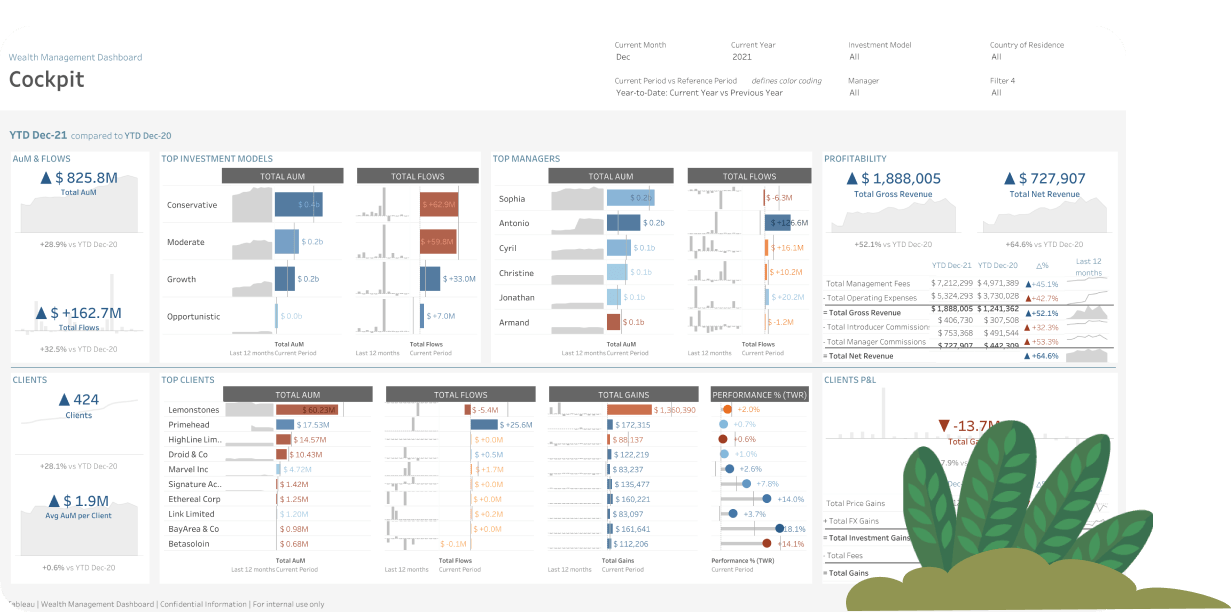This image is a Wealth Management Dashboard Cockpit displaying data for the Year-To-Date (YTD) figures as of December 21st, compared to YTD December 20th. At the top, the dashboard indicates a total wealth of $825.8 million with an upward arrow. Below that, there is another upward arrow showing $162.7 million. Further down, it lists 424 clients and $1.9 million in a net context. The center of the dashboard is filled with various colored lines and graphs, which are not legibly detailed but seem to encompass eight distinct graphs—four at the top and four at the bottom. 

On the right side, profitability is highlighted with figures showing a gross revenue of $1,888,005. The top right corner of the image details a total net revenue of $727,907. More writing is present that appears to provide additional insights, but it's too small to decipher clearly. At the very bottom of the image, there is a whimsical cartoon illustration of a plant.